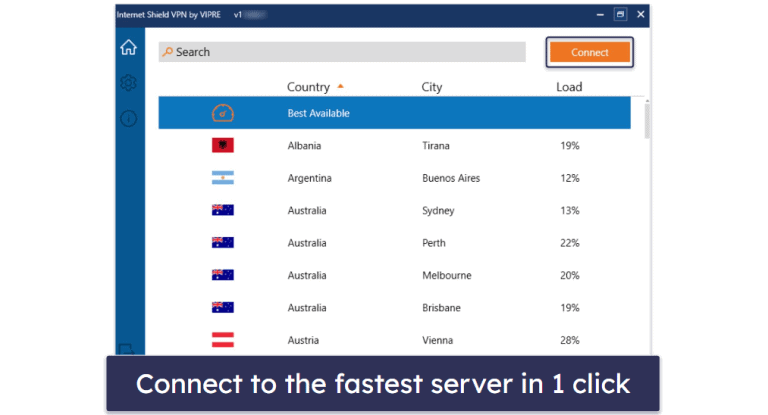This image displays a detailed interface of the Internet Shield VPN by VIPRE. At the top of the page, a navy blue banner spans horizontally, featuring the white text "Internet Shield VPN by VIPRE" on the left. To the right of the banner, three icons are displayed for minimizing, maximizing, and closing the window.

Running vertically along the left-hand side of the interface is a bright blue ribbon, prominently showing options labeled as "Home," "Settings," and "Help." The rest of the page is set against a white background, with a gray search box positioned at the top. Inside the search box, the text "search" is displayed alongside a gold-colored magnifying glass icon. To the right of the search box, an orange button labeled "Connect" in white letters is framed by a white border, which is further surrounded by a navy blue border.

The main content area of the page is organized into four vertical columns. The first column displays country flags, the second column spells out the names of the respective countries, the third column indicates the specific cities, and the fourth column shows the server load percentages. 

At the very bottom of the screen, a thick navy blue banner stretches across horizontally, with large white text urging users to "Connect to the fastest server in one click."